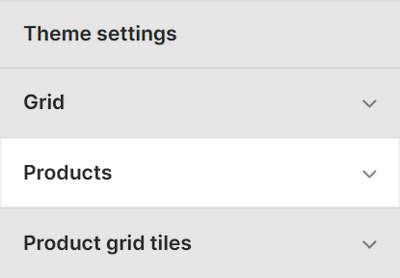A cropped screenshot displays what appears to be a mobile application's "Theme Settings" page. The header "Theme Settings" is prominently shown in a gray bar at the top. Below, three distinct options are available, each accompanied by a gray arrow, indicating the presence of drop-down menus. The first option is labeled "Grid" and presented in a gray bar. The second option, titled "Products," is set against a white bar. The third option, "Product Grid Tiles," appears within another gray bar. All text is rendered in a clear, black font. The layout and design bear a resemblance to interface elements found in mobile operating systems, possibly, though not definitively, of an Apple iOS nature. The image is tightly cropped, offering no additional context beyond these available selections.